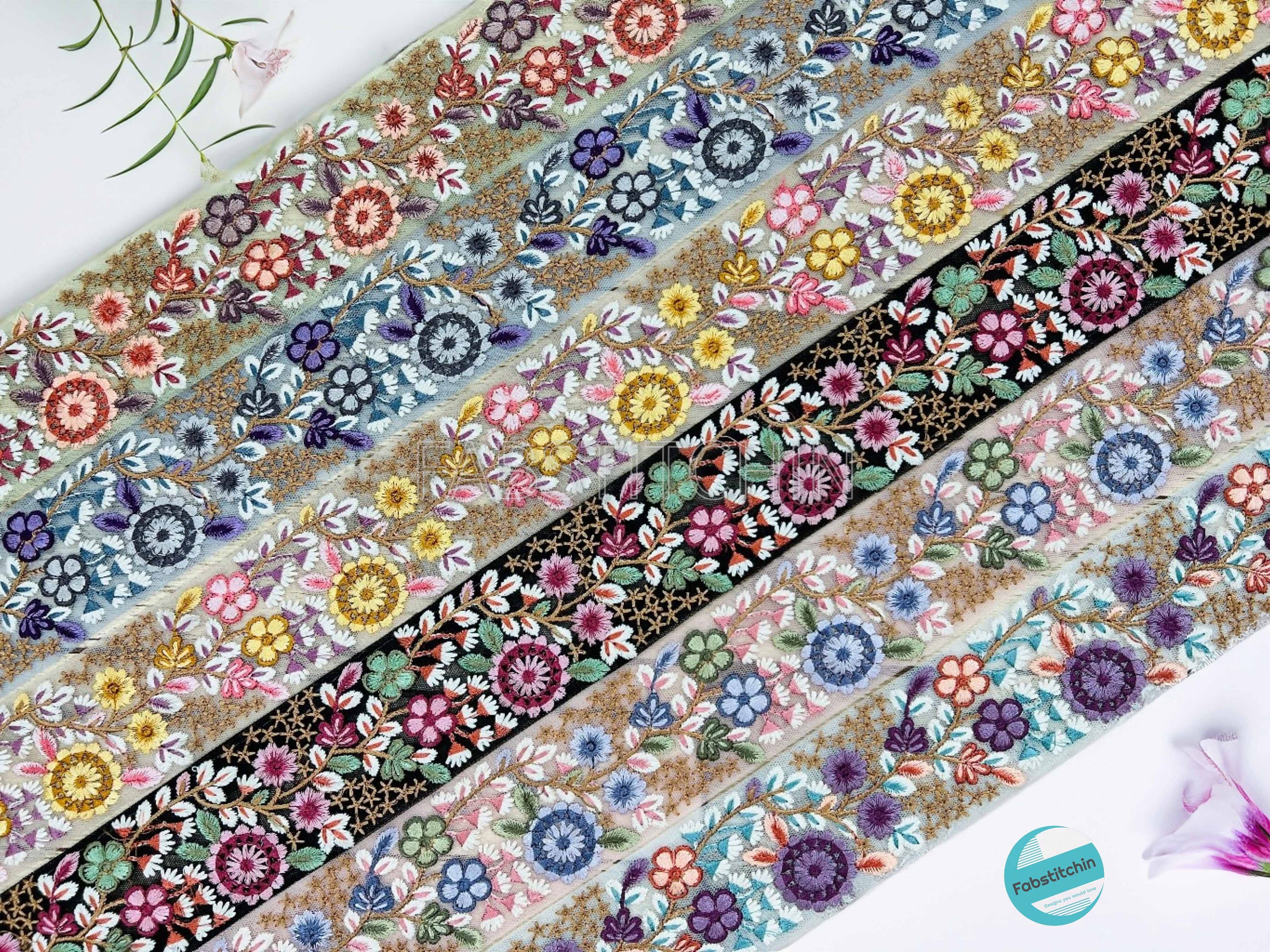The image showcases six diagonally arrayed fabric strips, positioned from the bottom left to the top right against a white background. Each strip features unique, detailed floral embroidery with vibrant colors and intricate patterns. These patterns include colors such as red, blue, yellow, purple, pink, orange, teal, light blue, green, and black, all adorned with brown stems and green leaves. The first strip on the top left is predominantly brown or orange with purple, the second is teal with light blue and purple, the third combines yellow, pink, and white, the fourth one is black with mauve and green, the fifth is blue with green and pink, and the last one features orange, beige, teal, and dark purple. Enhancing the aesthetics, a plant with green leaves and light pink flowers is placed diagonally opposite to the fabrics, positioned at the top left. At the bottom right, there's a circular logo that reads "fab stitching" in blue and white, accompanied by a small white and purple flower.